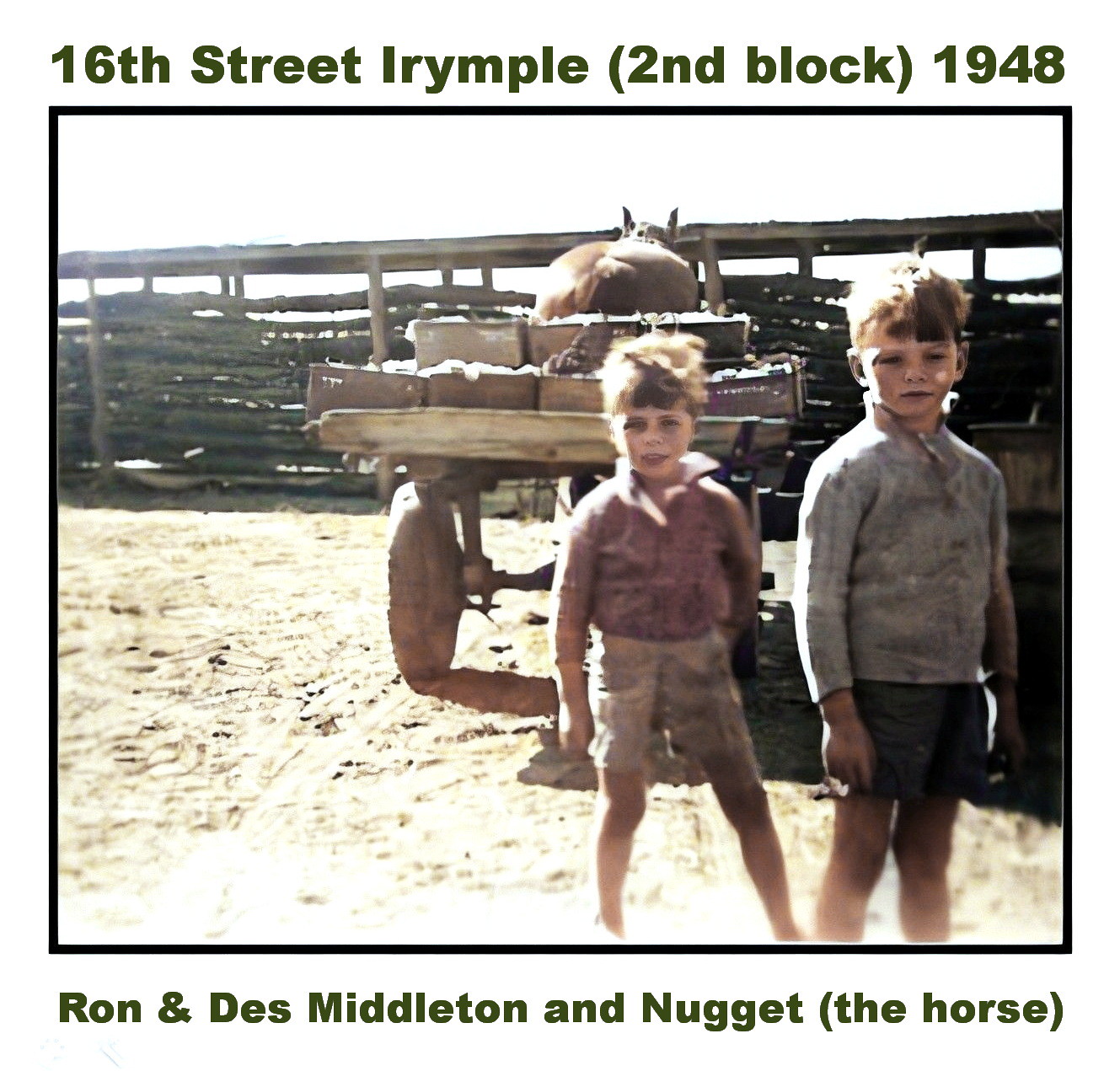This black-and-white photograph from 1948, titled "16th Street Irymple, 2nd Block," features two young boys, Ron and Des Middleton, accompanied by a large brown horse named Nugget. The image is framed by a white border with the text "Ron and Des Middleton and Nugget (the horse)" at the bottom. The boys, approximately 4 and 6 years old, appear to be on a farm, standing on a dirt ground with their knees visibly dirty. Both boys are dressed in long-sleeved shirts and shorts—one in a purplish shirt with grayish-blue shorts and the other in a blue shirt with dark shorts. They seem caught in a candid moment, gazing directly at the camera as if interrupted during their play or chores. Behind them, Nugget is harnessed to a wooden cart loaded with several wooden boxes, indicating farm work. The background depicts a rudimentary fenced area made from entire logs, likely part of a homestead structure, with a simple roofed section possibly used for animal transport. The entire scene under a white sky encapsulates a rustic, post-war rural life.